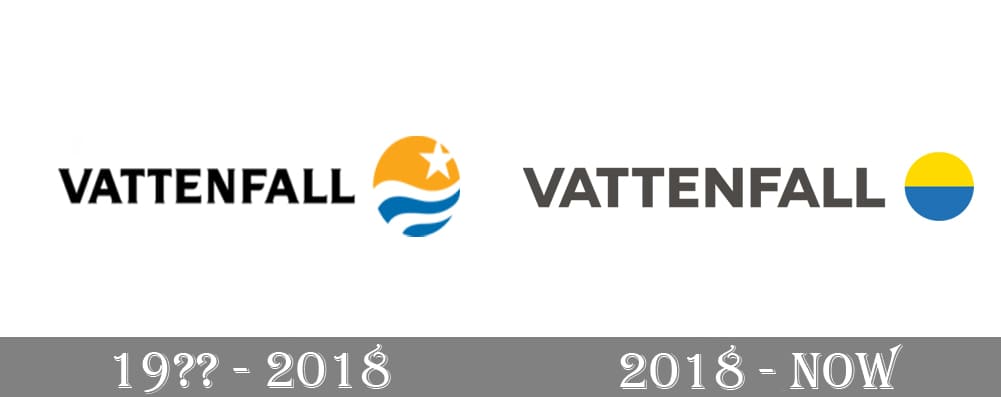The image is a promotional material for the company Vattenfall, highlighting their rebranding over time. The left half of the image shows the old Vattenfall logo set against a white background, with the years "19?? to 2018" displayed in white lettering within a gray bar. The old logo consists of a circle with a white star at the top, which is sandy-colored, representing sand, while the bottom part features alternating white and blue wavy lines symbolizing the sea. The word "Vattenfall" is depicted in black, all capital letters. The right half of the image displays the new Vattenfall logo, also set against a white background, showing the period "2018 to now" in white lettering within a gray bar. The new logo is a circle divided into two halves: the top half is yellow, and the bottom half is blue, similar to the colors of the Ukrainian flag. The name "Vattenfall" appears again in black capital letters, although in a slightly more grayish tone.